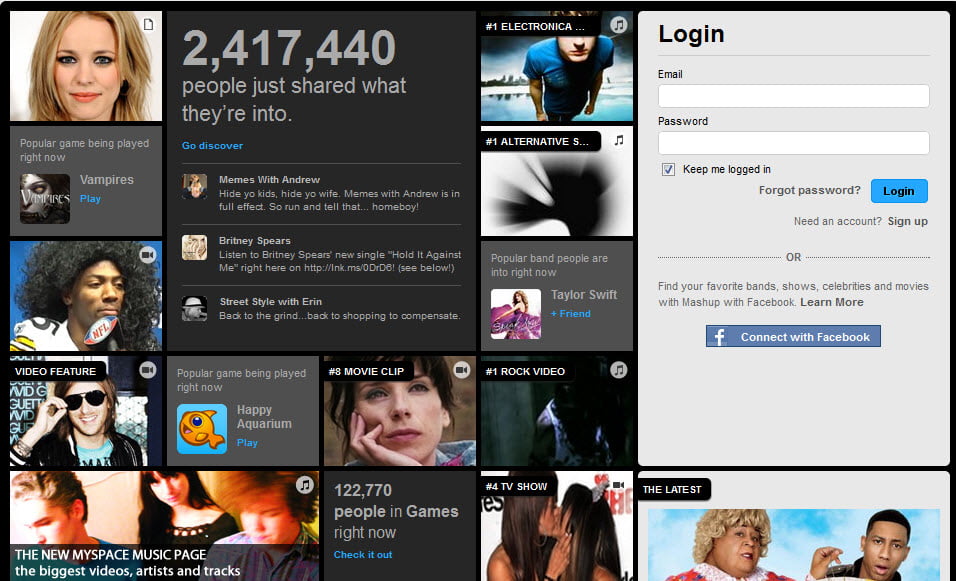The screenshot captures a bustling web page filled with a multitude of small photographs, graphics, and text boxes. Dominating the right-hand side is a prominent grey rectangle housing fields for email and password entry, enabling users to log in or sign up. This section also offers an option to connect via Facebook, facilitating seamless access. Surrounding this login module, various square and rectangular shapes pepper the page, each containing diverse content. Some showcase photos of people, while others feature small images accompanied by textual descriptions. Scattered hashtags, such as #movieclip, #rockvideo, and #TVshow, hint at the page’s multimedia offerings. In the bottom left-hand corner, a logo announces "The New MySpace Music Page," promising access to the latest and most popular videos, artists, and tracks.